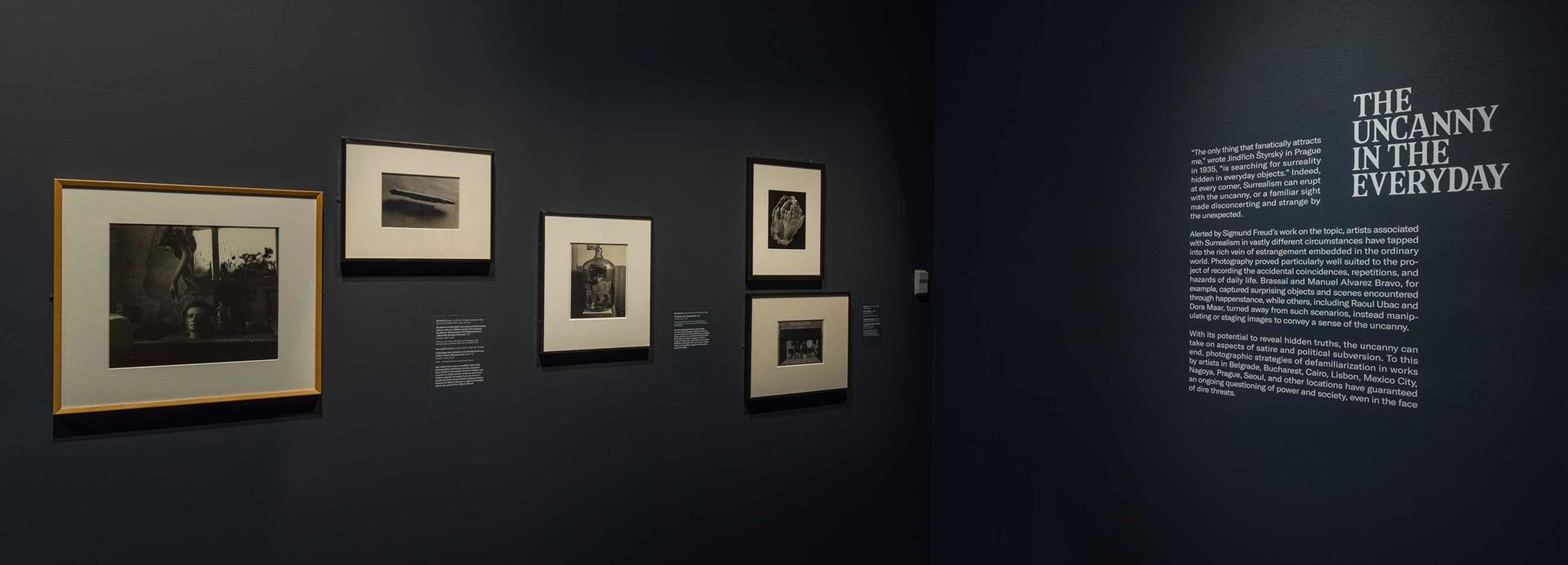The image depicts an art gallery interior with a visually striking setup. Dominating the scene is a long black wall on the left adorned with five framed photographs. The largest photo, positioned furthest to the left, is encased in a brown wooden frame and displays a black and white image featuring a woman’s face in a window. The other four photographs are in uniform black frames with white borders. The second photo appears to show a gray object resembling a missile atop an airplane, accompanied by small, unreadable white text. The third image consists of another black and white photograph, similarly featuring unreadable text nearby. The final two photographs are arranged vertically; the top one is taller and narrower with a yellow section, while the bottom is a square-shaped image in a black frame.

To the right of this gallery display, a shorter wall intersects at an angle, showcasing white text that reads "The Uncanny in the Everyday." Beneath this title, and to its side, are three paragraphs of explanatory text, though the specifics are too small to decipher from the image. The gallery space itself is painted entirely black, which contrasts sharply with the white lettering and framed photographs, enhancing their prominence and the overall mysterious ambiance of the exhibit. This meticulously arranged space suggests a thoughtful exploration of everyday scenes through an eerie and uncanny lens.